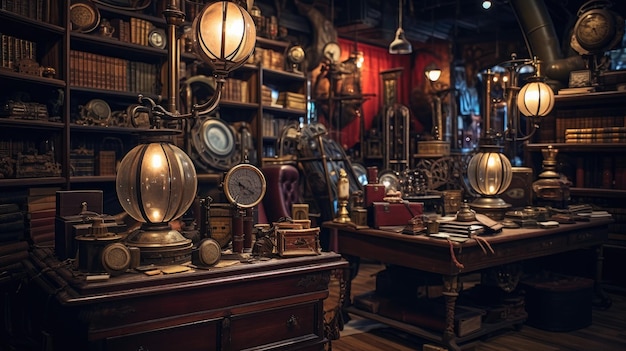The image depicts a detailed and intricately cluttered interior of a dimly-lit library or an office space, likely from a hidden objects video game. In landscape orientation, the digital drawing presents a rich steampunk aesthetic, merging old-world charm with futuristic elements. The room is dominated by an array of dark wooden bookcases overflowing with books, flanked by large brown desks cluttered with various items, boxes, and knickknacks. Illuminating the scene are numerous lanterns and futuristic but antiquated-looking lamps, casting a warm yellow glow throughout the room.

A striking red curtain hangs from the ceiling at the top center, adding a touch of bold color amidst the predominantly drab hues of browns, yellows, and golds. To the right of the curtain, a burst of light blue illuminates several objects, enhancing the mysterious ambiance. On the right side of the room, a bookcase holds a clock on its top shelf, with more light blue light dispersing above and slightly to the left of it. The middle and foreground of the scene feature tables piled with books, lamps, and an assortment of gadgets and doodads, contributing to the cluttered yet fascinating setting. The absence of people and text in the image emphasizes the evocative atmosphere of this seemingly alchemical, and curiously chaotic, library.